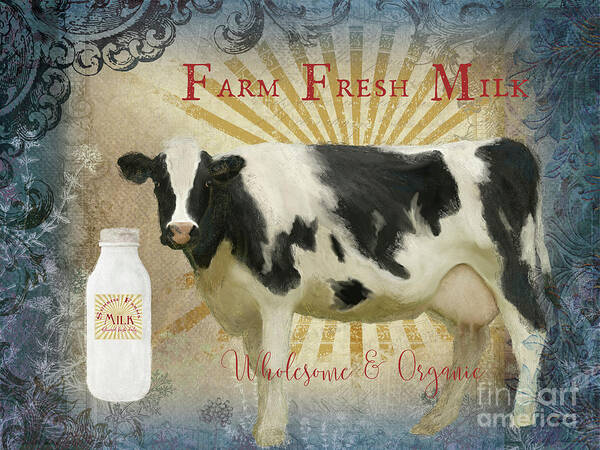The image is a detailed, picturesque portrayal of a black and white dairy cow, positioned at the center with its face looking directly at the viewer and light pink udders visible. Surrounding the cow is a vibrant yellow sunburst background, with highly detailed red lines emanating, giving an effect of the sun shining brightly behind the cow. At the top of the image, “FARM FRESH MILK” is prominently displayed in bold, capitalized, red serif letters, providing an old-fashioned charm. Below the cow, the words “Wholesome and Organic” are inscribed in a playful, whimsical cursive font, adding a feminine and fun touch to the presentation. Framing the whole image, there's an ornate border featuring darker blue hues and elegant scrollwork, evoking the look of gilded frames from antiquity. 

To the left of the cow, a white glass milk jug with a beige lid can be seen, bearing the same starburst logo with yellow in the center and the word “MILK” inscribed in bold, capitalized red letters. The corners of the image are adorned with additional floral or herbal designs, enhancing the vintage aesthetic. In the bottom right corner, there is text, “fine art america,” adding a mark of identity to the piece.